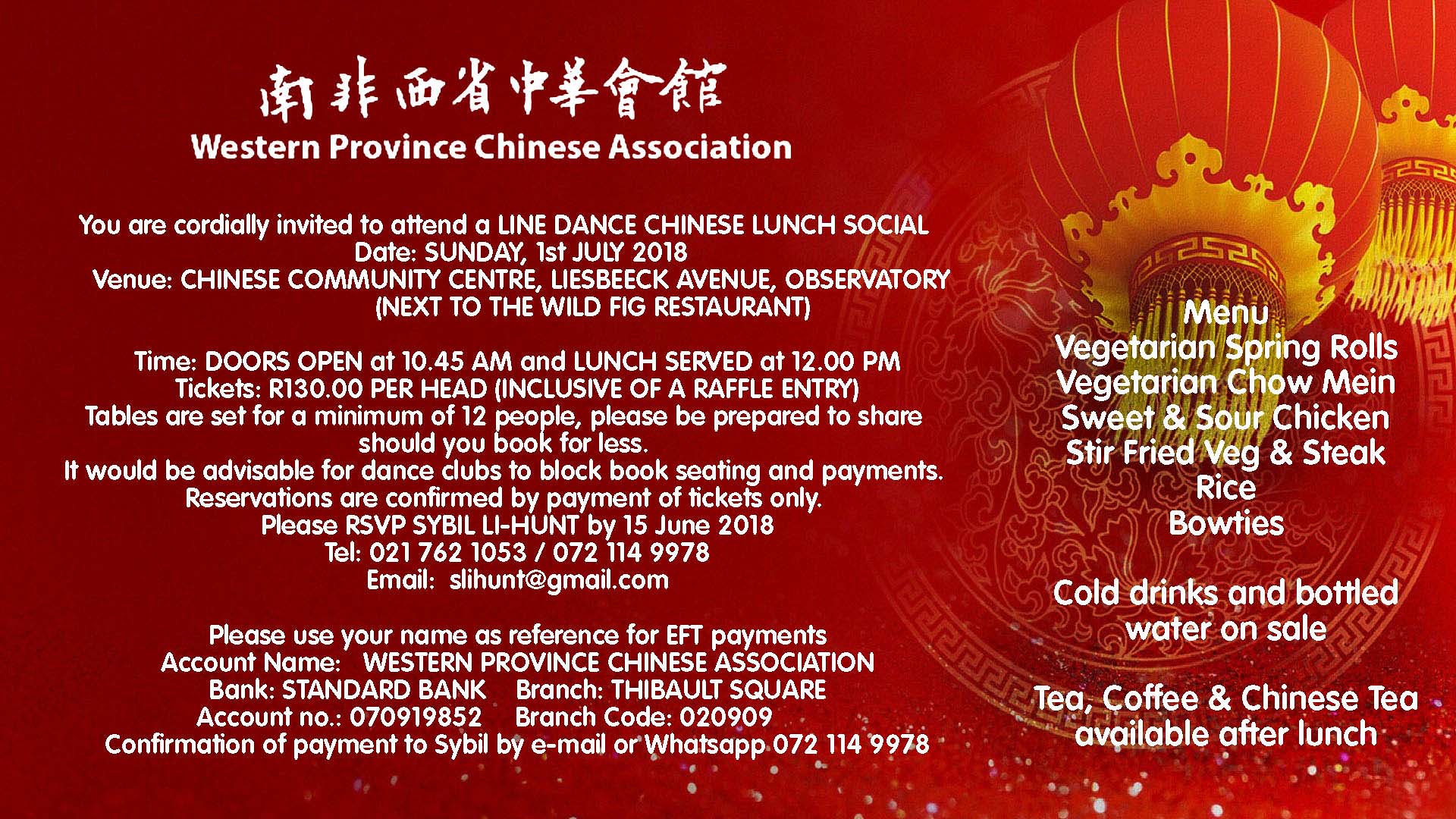A leaflet advertising a social event hosted by the Western Province Chinese Association. The background transitions from a pretty purple color on the left side to a lighter orange on the right, with golden balloons featuring yellow tassels floating upwards in the upper right corner. At the top left, there are Chinese characters followed by the text "Western Province Chinese Association." You are cordially invited to attend a Lion Dance Chinese Lunch Social. 

**Date:** Sunday, 1st July 2018  
**Venue:** Chinese Community Center, Leisbeck Avenue, next to the Wild Fig Restaurant.  
**Time:** Doors open at 10:45 a.m., lunch served at 12 p.m.  

**Tickets:** R130.00 per head, inclusive of a raffle entry. Tables are set for a minimum of 12 people; please be prepared to share should you book for less. Dance clubs are advised to block book seating and make payments accordingly. Reservations are confirmed by payment of tickets only.

**RSVP:** Sybil Li-Hunt by 15th June 2018  
**Telephone:** 021-762-1053 / 072-114-9978  
**Email:** slihunt@gmail.com  

Please use your name as a reference for EFT payments.  

**Account Information:**  
- **Account Name:** Western Provincial Chinese Association  
- **Bank:** Standard Bank  
- **Branch:** Tygerberg Square  
- **Account Number:** 070919852  
- **Branch Code:** 020909  

Confirmation of payment can be sent to Sybil by email or WhatsApp at 072-114-9978.

On the right side of the leaflet, the menu lists: Vegetarian spring rolls, vegetarian chow mein, sweet and sour chicken, stir-fried vegetables, and steak rice, with brownies for dessert. Cold drinks and bottled water are for sale, and tea, coffee, and Chinese tea will be available after lunch.